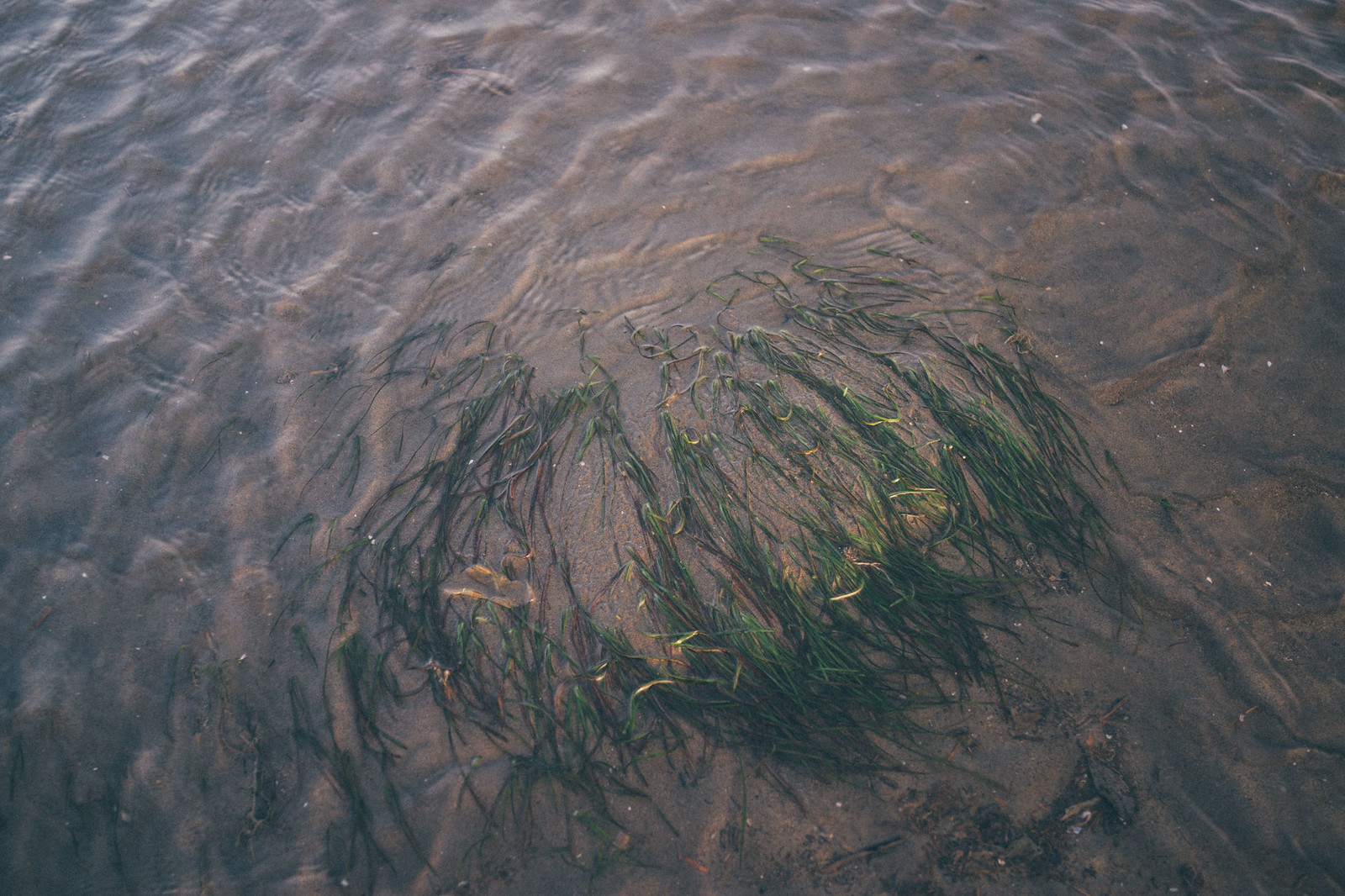This color photograph, taken outdoors during the daytime, captures a unique and artistic scene that is likely situated by a beach. Dominating the visual is a rich, dark brownish expanse that could either be shallow water or an unusual shade of sand. This surface is marked with numerous small ripples and waves, contributing to a textured, dynamic appearance.

At the center of the composition, a small cluster of green grass or sea vegetation stands out. The grass appears to be laying on its side, either floating on the water or resting on the sand. Surrounding this area, the water—or sand—features tiny ripples, indicating a shallow environment. The refraction of light through the shallow water further enhances the intricate details of the sandy or watery foreground. This intriguing interplay of natural elements suggests a captivating, shallow coastal scene, blending water, sand, and vegetation harmoniously.